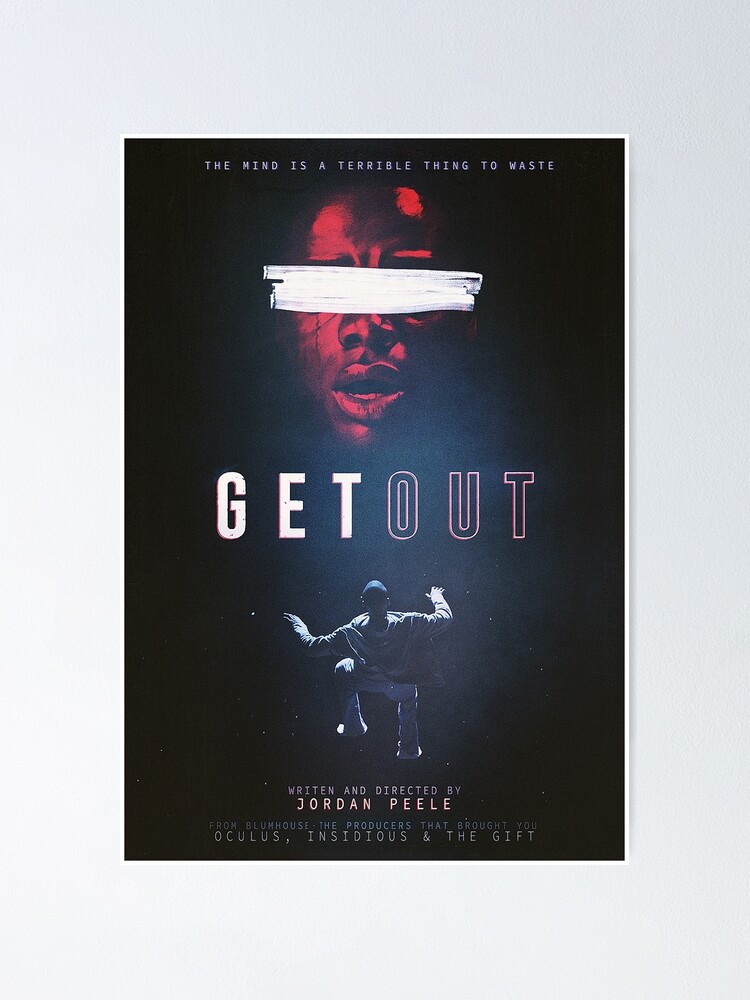A captivating poster set against a white wall showcases the film "Get Out." The poster itself is a vertical rectangle with a thin white border, predominantly featuring a black background. At the top of the poster, a quote in white capital text reads, "The mind is a terrible thing to waste." Below this, a man's face, illuminated in red, conveys fear as a white strip obscures his eyes. Centered in the poster, the title "Get Out" is prominent; "Get" is bold and white while "Out" is outlined in pink. Mid-poster, there is another striking image of a man, arms outstretched and leg lifted, seemingly caught in mid-leap, dressed in white. Below this, the text reads, "Written and Directed by Jordan Peele" and includes the production credits: "From Blumhouse, the producers that brought you Oculus, Insidious, and The Gift." The fusion of these elements creates a stark, dramatic visual, characteristic of poster art.